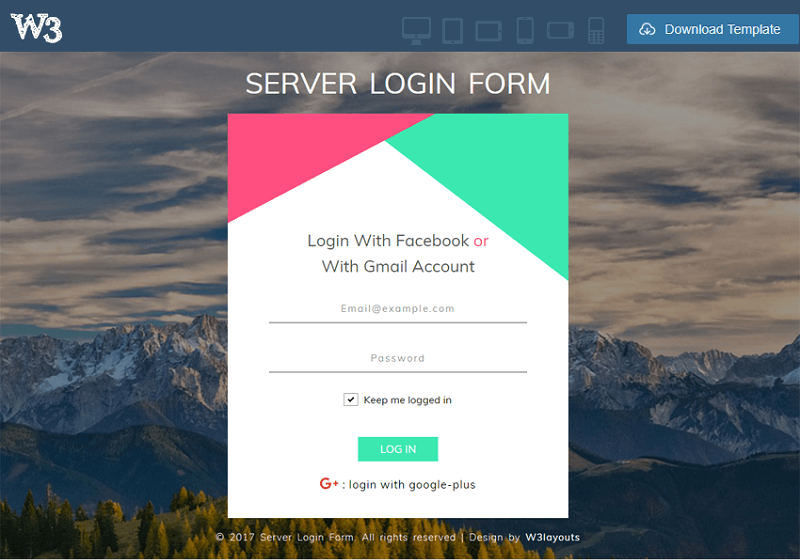This image is a screenshot from a website, which features a prominent blue bar at the upper left-hand corner displaying "W3." Below this bar, the main visual element is a photograph depicting a serene mountain landscape. Overlaying this picturesque scene is a translucent window labeled "Server Login Form."

Within the Server Login Form, users are presented with multiple login options. The form offers the ability to log in using either a Facebook account or a Gmail account. For those opting to manually enter their credentials, the form provides designated fields: one for the email address at the top and another for the password directly below it. Additionally, there is a checkbox labeled "Keep me logged in" that users can select for convenience.

At the bottom of the form, a prominent green login button invites users to submit their credentials. Alternatively, there is an option to log in using a Google+ account, clearly marked as clickable text for easy access. 

Overall, the screenshot effectively combines aesthetics with functionality, incorporating a beautiful background image with an intuitive login interface.